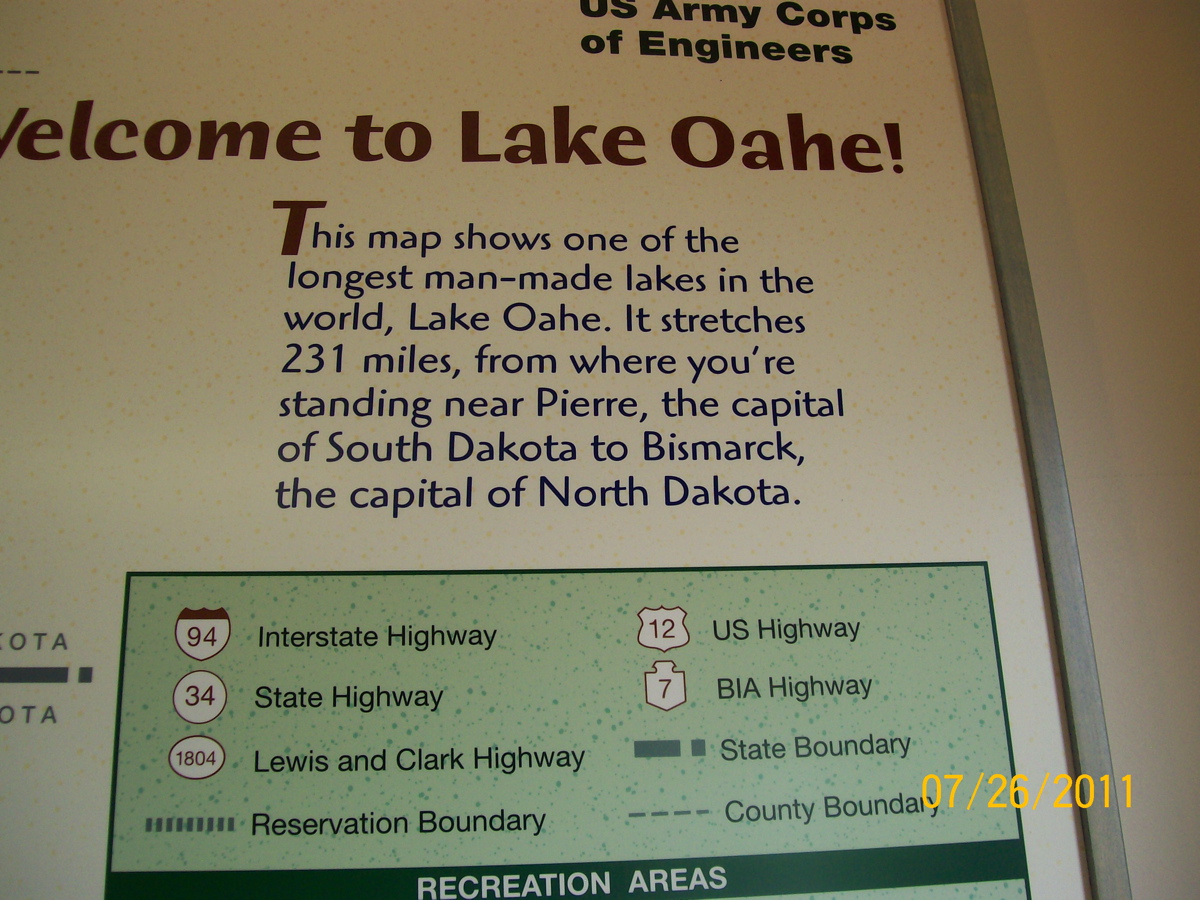This is a detailed close-up color photograph of a section of an informational map sign. Prominently, at the top right corner, it reads "U.S. Army Corps of Engineers" in black text. Below that, in brown text, the sign welcomes you with "Welcome to Lake Oahe, O-A-H-E!" The paragraph that follows provides informative details, stating: "This map shows one of the longest man-made lakes in the world, Lake Oahe. It stretches 231 miles from where you're standing near Pierre, the capital of South Dakota, to Bismarck, the capital of North Dakota." 

Beneath this descriptive paragraph, there is a green rectangle containing a map key, which although the map itself is not visible, includes various symbols and their meanings. The key lists: 94 Interstate Highway, 34 State Highway, 1804 Lewis and Clark Highway, 12 U.S. Highway, 7 BIA Highway, and denotes a Reservation Boundary with small green lines, a State Boundary with large green lines, and a County Boundary with skinny dotted lines. The section also includes another segment indicating "Recreation Areas" in a darker green box. The date, "07-26-2011," is also marked on the sign, giving it a historical context. The entire setup is akin to a placard you might find upon arriving at a significant recreational site or natural attraction like Lake Oahe.